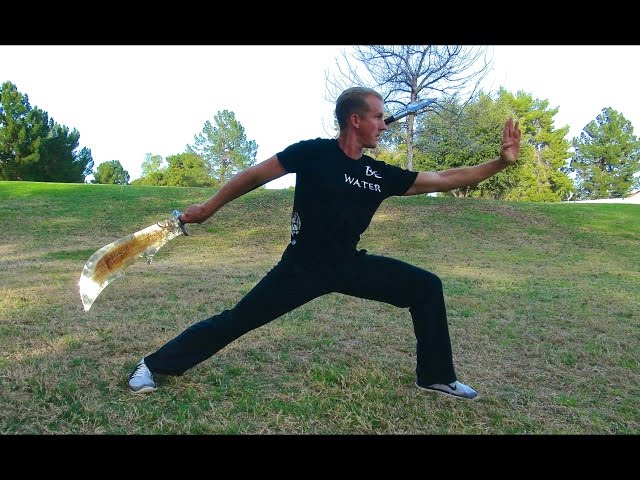In the image, a middle-aged man with tan skin and brown hair is deeply engaged in a martial arts practice, striking a dramatic, lunging karate stance. He is situated in a verdant park with well-manicured green grass, under a clear sky. Behind him, a mix of trees includes tall evergreens and a single, bare deciduous tree. The man wears a black short-sleeve t-shirt emblazoned with a design that includes the word "water," along with black slacks and light blue athletic shoes. His right hand wields a large, gleaming silver sword that is almost leg-length, featuring a stylish brown grip or embellishment. His left hand is extended forward, fingers splayed. The overall scene suggests a serene, sunny day, embodying both the discipline of martial arts and the tranquil beauty of nature.